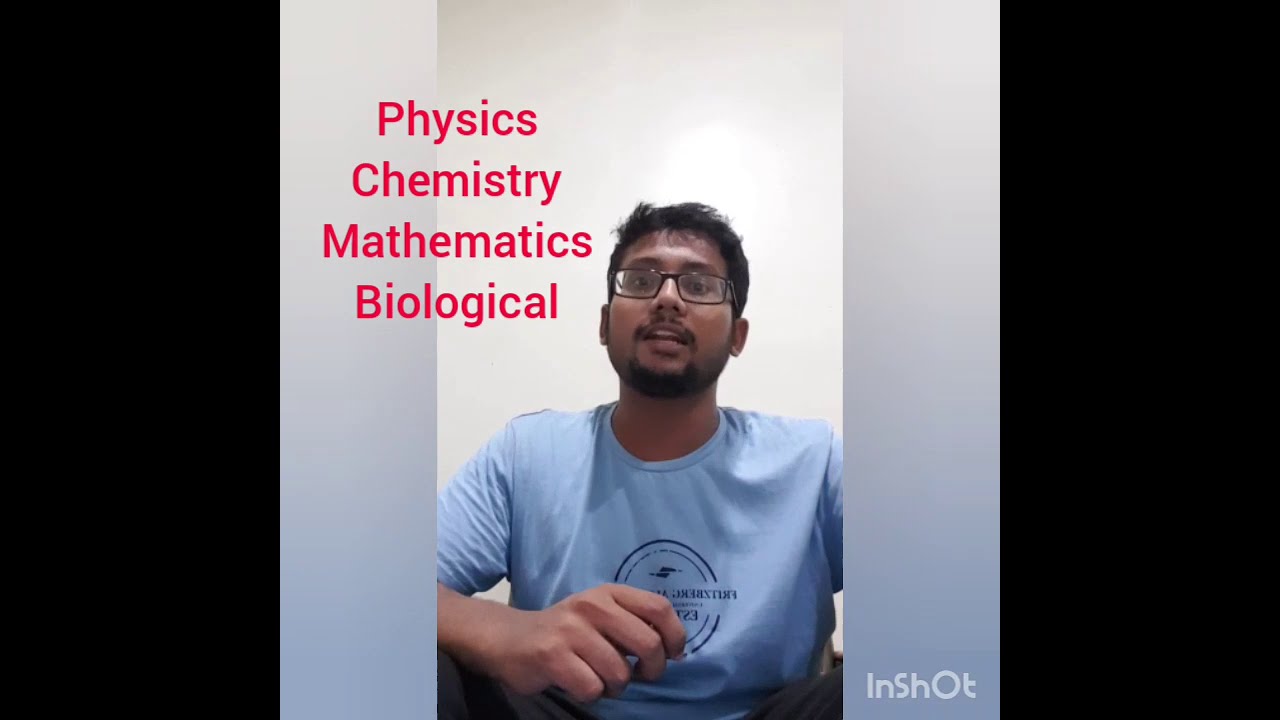The image captures a medium-skinned gentleman with short, black hair and a dark goatee, wearing rectangular eyeglasses. He is dressed in a blue T-shirt featuring a circular design and possibly wearing khaki pants. The man is positioned against a divided background with two vertical banners fading from white to bluish, one on each side. These banners are flanked by black strips on the far left and right edges. The man, seated in the center with one arm angled forward, appears to be engaged in a webcast. Behind him, the background is white, and there is red text above his right shoulder that reads “Physics, Chemistry, Mathematics, Biological." Additionally, the bottom-right corner of the image displays the word "InShot" in white text. The overall setting gives the impression of the man being boxed in between two walls, partially obscuring parts of his arms.